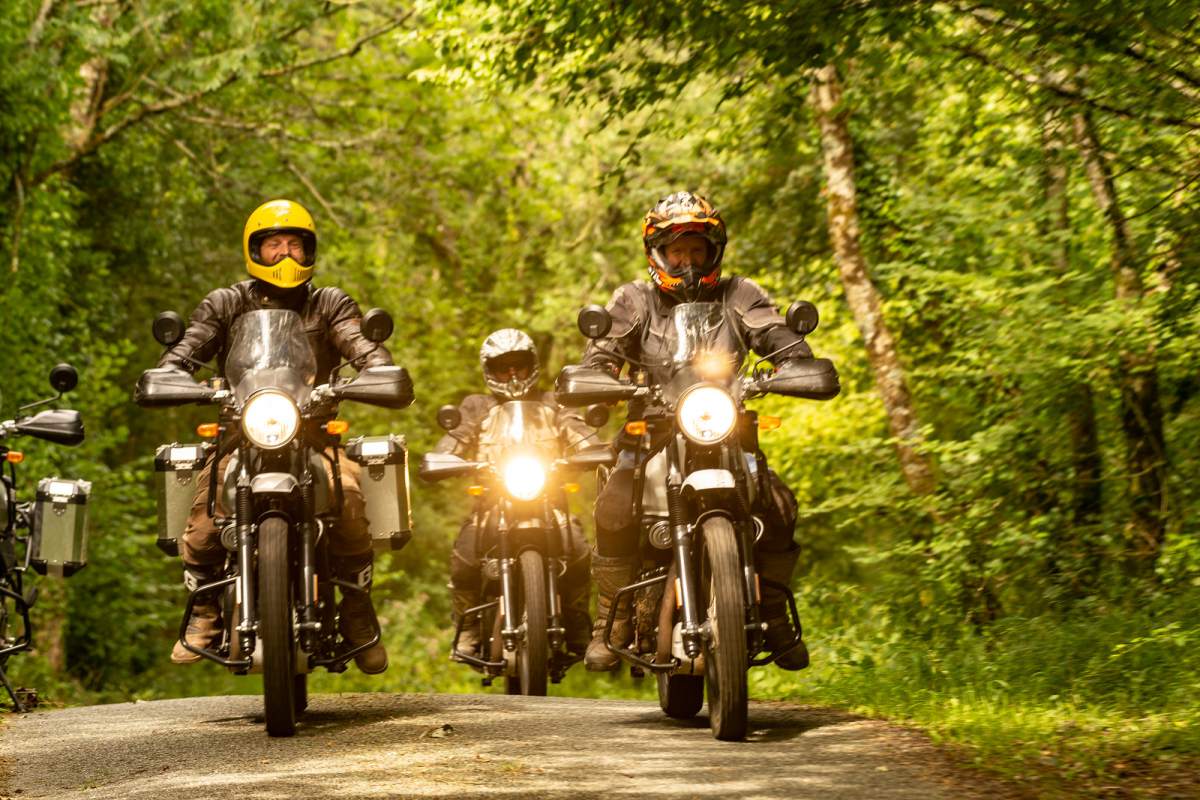In this detailed outdoor photograph taken during daylight, three motorcyclists are prominently featured riding towards the camera, their bright headlights shining directly at the viewer. They travel on a black or gray asphalt road winding through a forest, flanked by lush green trees. Each rider wears protective leather clothing and a helmet: the motorcyclist on the left sports a yellow helmet and has a baggage compartment on the back of their large displacement street bike, suggesting some off-road activity; the rider in the center, positioned slightly behind the others, is in a white helmet and black attire; and the motorcyclist on the right wears an orange and black helmet. Boots complete their gear as they navigate the scenic and well-lit forest road. The colors in the image are vivid, with a mix of greens, browns, blacks, and grays, capturing the essence of motorcycling through the wilderness.